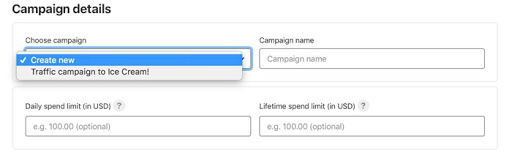The image features a form layout set against a white background. In the upper left corner, there is black text that reads "Campaign Details." Below this heading is a gray-lined box containing gray text that says "Choose Campaign," accompanied by a pull-down menu. When activated, the pull-down menu reveals a blue banner with white text that says "Create New," along with a check mark symbol.

Beneath this section, inside the same box, there is black text describing a traffic campaign related to ice cream. Additional text specifies "Daily Spend Limit in USD: $100" with the note "optional."

In the upper right corner of the image, there is another gray box with black text that reads "Campaign Name." Below this, situated right above another gray box, it says "E.g., $100 optional." The second gray box is headed by black text that reads "Lifetime Spend Limit in USD."